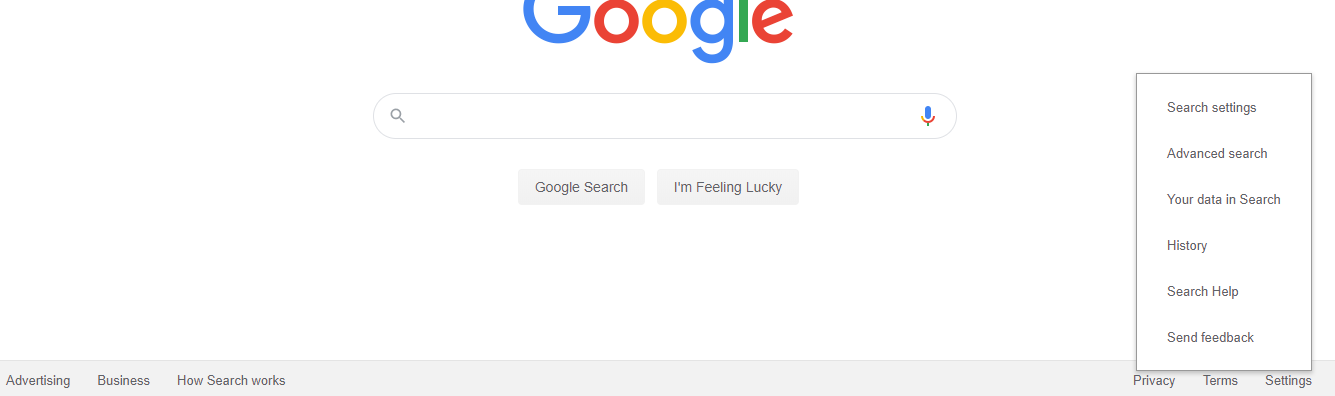A screenshot captures a partial view of the Google homepage, with its iconic, multicolored logo at the top. The capital "G" in blue, the first lowercase "o" in red, second "o" in yellow, "g" in blue, "l" in green, and "e" in red are visible, but the tops of the capital "G" and lowercase "l" are cut off due to an incomplete zoom on the webpage. Below the logo, the familiar white search bar is centered, featuring a blue-tipped microphone icon inside it. Two buttons are prominently displayed underneath: one labeled "Google Search" and the other "I'm Feeling Lucky."

To the right side of the search bar, a narrow, vertical white rectangle with a gray border is open, revealing a menu. This menu lists several options in a vertical arrangement: "Search settings" at the top, followed by "Advanced search," "Your data in search," "History," "Search help," and finally, "Send feedback." Additional clickable items are also listed in a line below this menu.